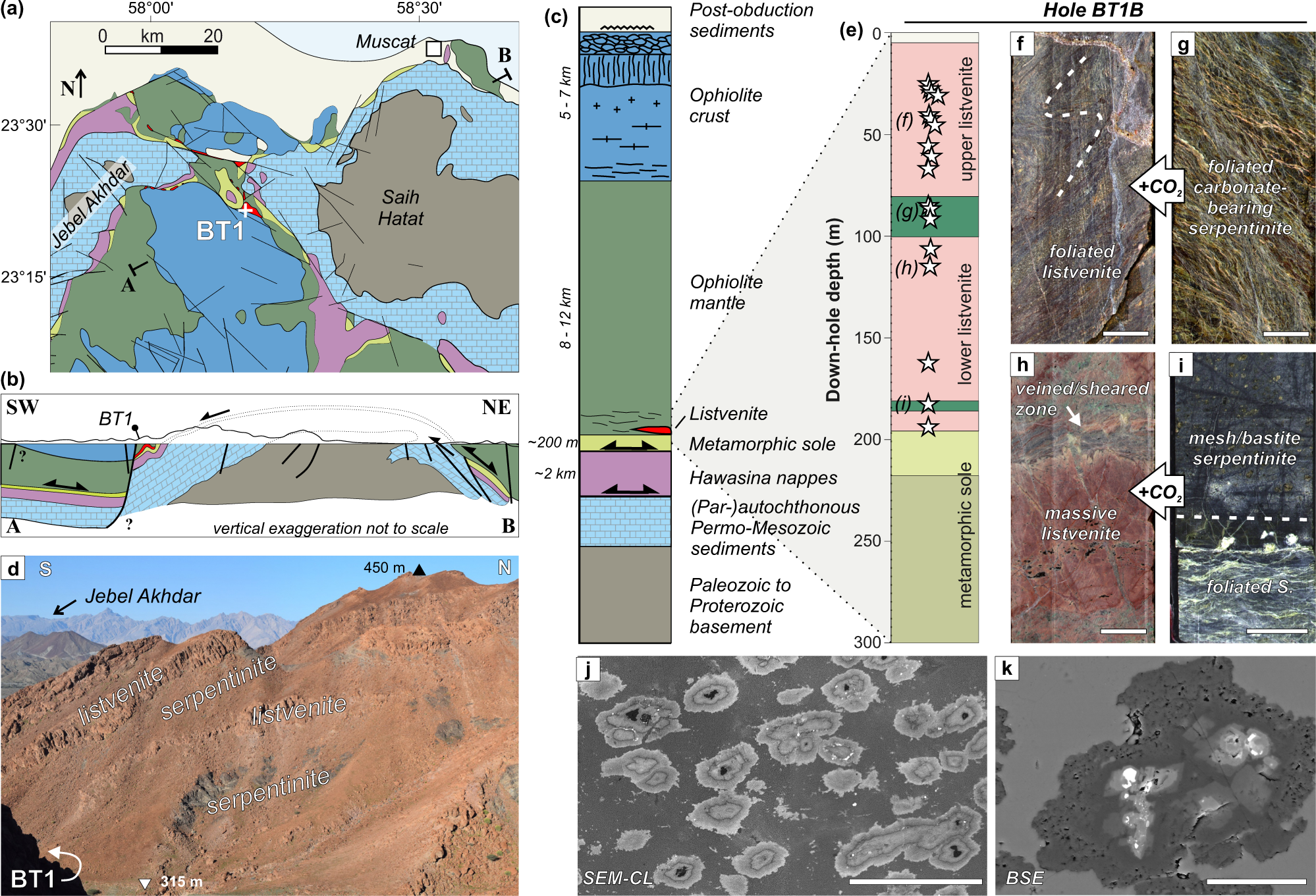The image is a detailed poster featuring ten different maps and diagrams that illustrate various geological and geographical features. The top-left map displays different colors representing various terrains, including bodies of water, and uses textbook-style illustrations. Below it are a small square map and a mountain illustration, likely indicating specific locations related to the top map. The map to the right contains unreadable text but appears to continue the theme of geographical representation. Beneath this is a grayish-brown map with circles and dots, possibly indicating geological formations. On the right, there are four equally-sized square maps that are somewhat blurry, followed by another grayish-black map with white dots in the middle, suggestive of geological data points.

Central to the poster is text describing "post-abduction sediments" and a detailed graph that charts different sedimentary layers, including "Gisventite," "Serpentinite," "Ophelia crust," and "Ophiolite mantle," among others. This central section provides a cross-sectional view of sedimentary layers ranging from the Ophelite crust to the Paleozoic to Protozoic basement. The right side of the poster includes explanatory images and maps that highlight where these geological components can be found. Overall, the poster appears to be a comprehensive depiction of different geological and geographical elements, combining both illustrative maps and real-time images to convey detailed scientific information.